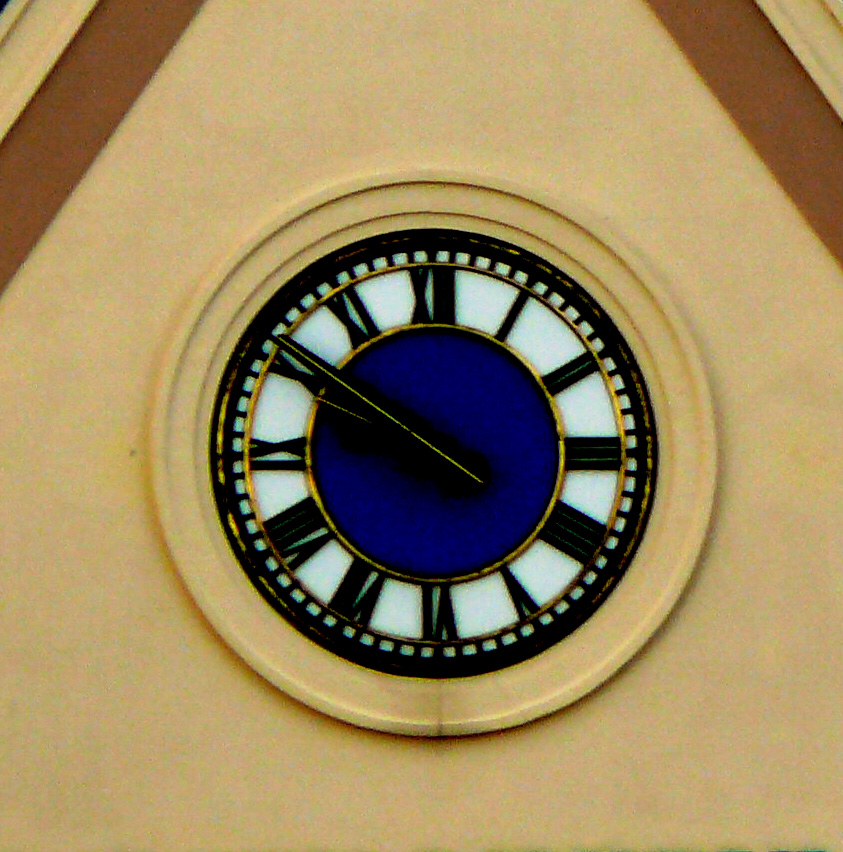This detailed photograph captures a classical clock embedded within the stone wall of a building. The wall surrounding the clock is a light yellow or cream color, with small brown lines extending from the top left and right edges, which likely represent the edges of an awning or other structural element, giving a triangular shape to the surrounding space. The clock has a black outer border from which small black lines extend inward toward a gold-bordered clock face adorned in white or transparent glass, showcasing black Roman numerals from I to XII. Inside this perimeter is another gold border encircling a dark green or blue central area. The clock's hands are black with a gold stripe running down their middle, positioned to indicate the time. Although the image is zoomed in on the clock face, the triangular form and the architectural detail suggest the clock is mounted on the exterior upper section of the building, potentially resembling a stained glass window.